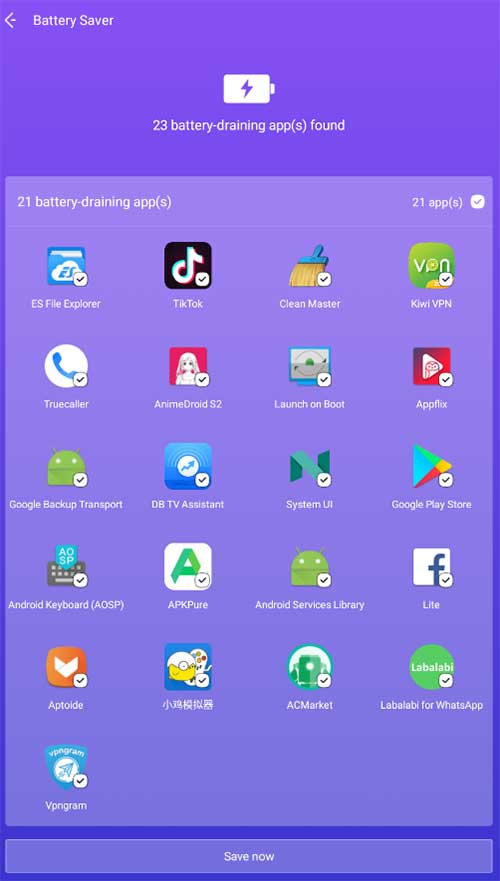The image depicts a screenshot of a device settings page, likely from a mobile phone or laptop, featuring a light purple background. At the top left corner, white text reads "Battery Saver," accompanied by a left-pointing white arrow. Centrally located below is an icon of a white battery silhouette with a purple lightning bolt inside it.

Under the icon, the text states, "23 battery draining apps found." Following this, a new section begins with "21 battery draining apps" on the left and "21 apps" with a check mark on a white background on the right.

This section lists various app icons horizontally:
1. ES File Explorer
2. TikTok
3. Clean Master
4. Kiwi VPN

Below, the next row includes:
1. Truecaller
2. Anime Droid S2
3. Launch on Boot
4. AppFlix

The subsequent row features:
1. Google Backup Transport
2. DBTV Assistant
3. System UI
4. Google Play Store

Further down are:
1. Android Keyboard (AOSP)
2. APK Pure
3. Android Services Library
4. Lite

The final row lists:
1. Aptoide
2. An app with a Japanese name
3. AC Market
4. ABI for WhatsApp

At the very bottom, to the left, it reads "VPN Grasm" or "VPN Gram," again with white text on a light purple background. A rectangular button spans the width of the screen at the bottom center, with "Save Now" written in white text.